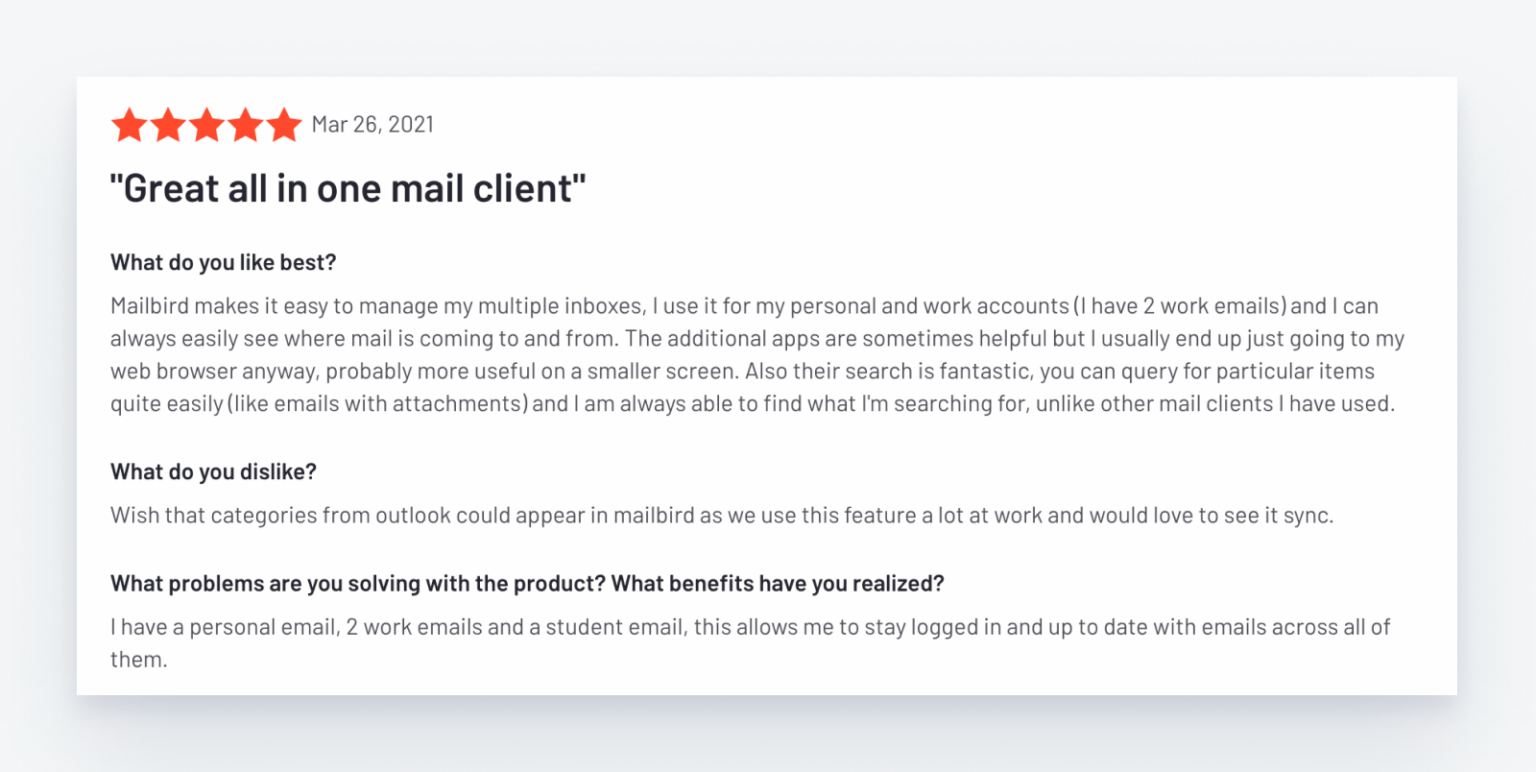The image captures a screenshot of a detailed user review for a mail client called Mailbird. 

The review is displayed within a long rectangular white box, set against a light gray background with a border. In the upper left corner, there is a set of five orange stars indicating the rating. To the right of the stars, it shows the review date: March 16th, 2021. 

Beneath the date, in a black header format, the title of the review reads, "Great All-in-One Mail Client." Below this, another header in bold black text asks, "What do you like best?" The user's response is provided in lighter text: "Mailbird makes it easy to manage my multiple inboxes. I use it for my personal and work accounts (I have two work emails), and I can always easily see where my mail is coming to and from. The additional apps are sometimes helpful, but I usually end up just going to my web browser anyway—probably more useful on a smaller screen. Also, their search is fantastic. You can query for particular items quite easily (like emails with attachments), and I'm always able to find what I'm searching for, unlike other mail clients I have used."

Following this, another bold header poses the question, "What do you dislike?" The reviewer's answer, also in light text, notes: "Wish that categories from Outlook could appear in Mailbird as we use this feature a lot at work and would love to see it sync."

Finally, another section begins with a bolded header asking, "What problems are you solving with this product? What benefits have you realized?" The response, in regular text, reads: "I have a personal email, two work emails, and a student email. This allows me to stay logged in and up to date with emails across all of them."